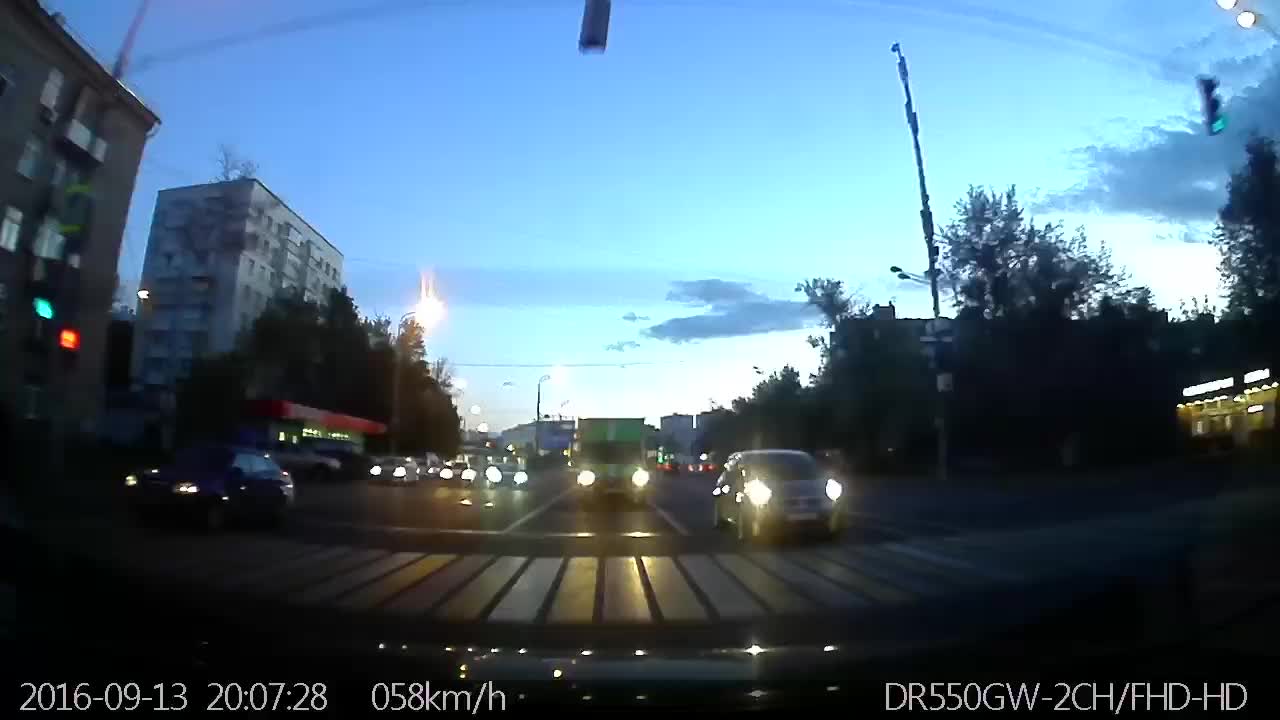The image is a realistic photograph taken from the perspective of a car, possibly from a dash cam or rear view mirror, during the early evening or late morning as indicated by the dark blue sky and the setting or rising sun casting long shadows on the street. The scene shows an urban environment with heavy traffic, featuring several cars with their headlights on, including a noticeable green truck among smaller vehicles. The street is marked with white lines and includes a visible crosswalk immediately behind the car. On the left side, two large buildings, likely apartments given their concrete structure and numerous windows and balconies, frame the scene. Meanwhile, the right side of the image shows another lit-up building. Traffic lights indicating green are visible towards the top of the image. The photograph is timestamped with white text at the bottom: "2016-09-13 20:07:28 058 km/h" on the left, and "DR550GW-2CH/FHD-HD" on the right.